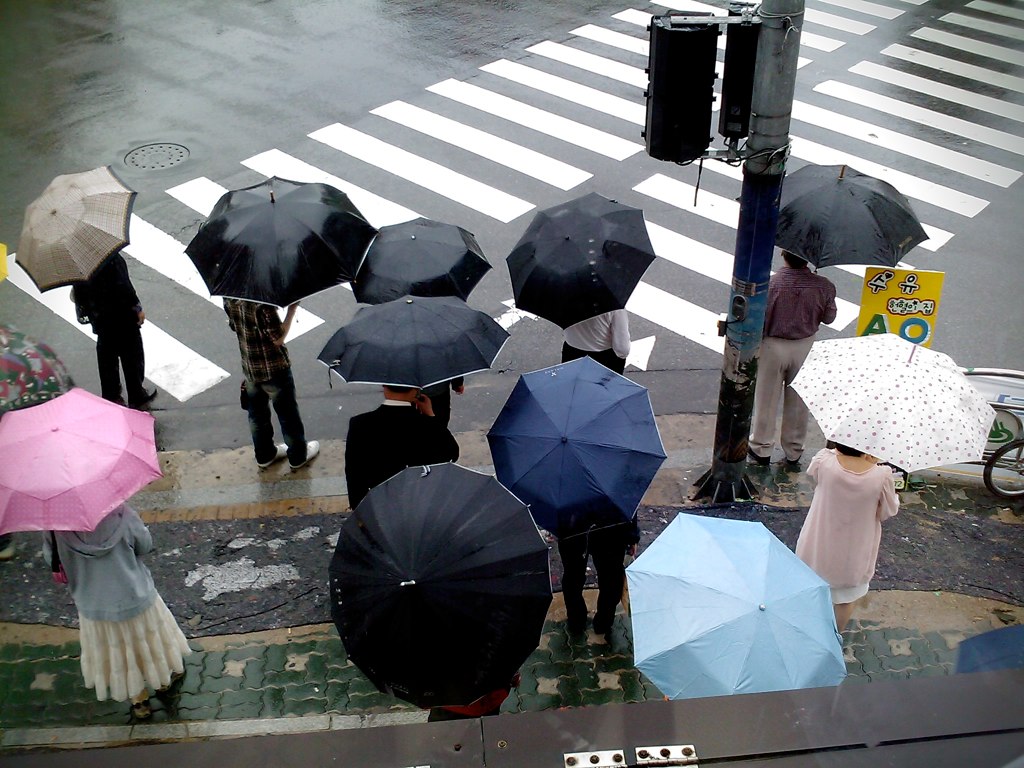This photograph captures a rainy day at a pedestrian crossing, likely in Japan, given the small yellow sign with Japanese characters visible on the street. Featuring a bird's-eye view from an elevated angle, the image shows a large, double-stripe zebra crossing in front of a group of people on a wet sidewalk. The pedestrians, mostly viewed from behind, hold a variety of umbrellas while waiting to cross—black being the most common color. Notably, a woman in a long white skirt and a bluish-grey tracksuit top holds a pink umbrella on the left side, alongside another woman on the right with a white umbrella adorned with pink and bluish dots and dressed in a pink shirt or gown. Other distinctive umbrellas include a light blue, a dark blue, and a sandy-colored one. The crowd also features men and women in dark clothing, except for one person wearing a red shirt and khaki pants. The multi-colored brick sidewalk, consisting of green, gray, black, and sandy-colored bricks, adds texture to the scene, and you can spot the wheel of a bicycle on the right side. The rainy atmosphere is accentuated by the wet surfaces of the road and sidewalk, further enhanced by the reflections and the people's posture as they wait under their umbrellas for the light to change.